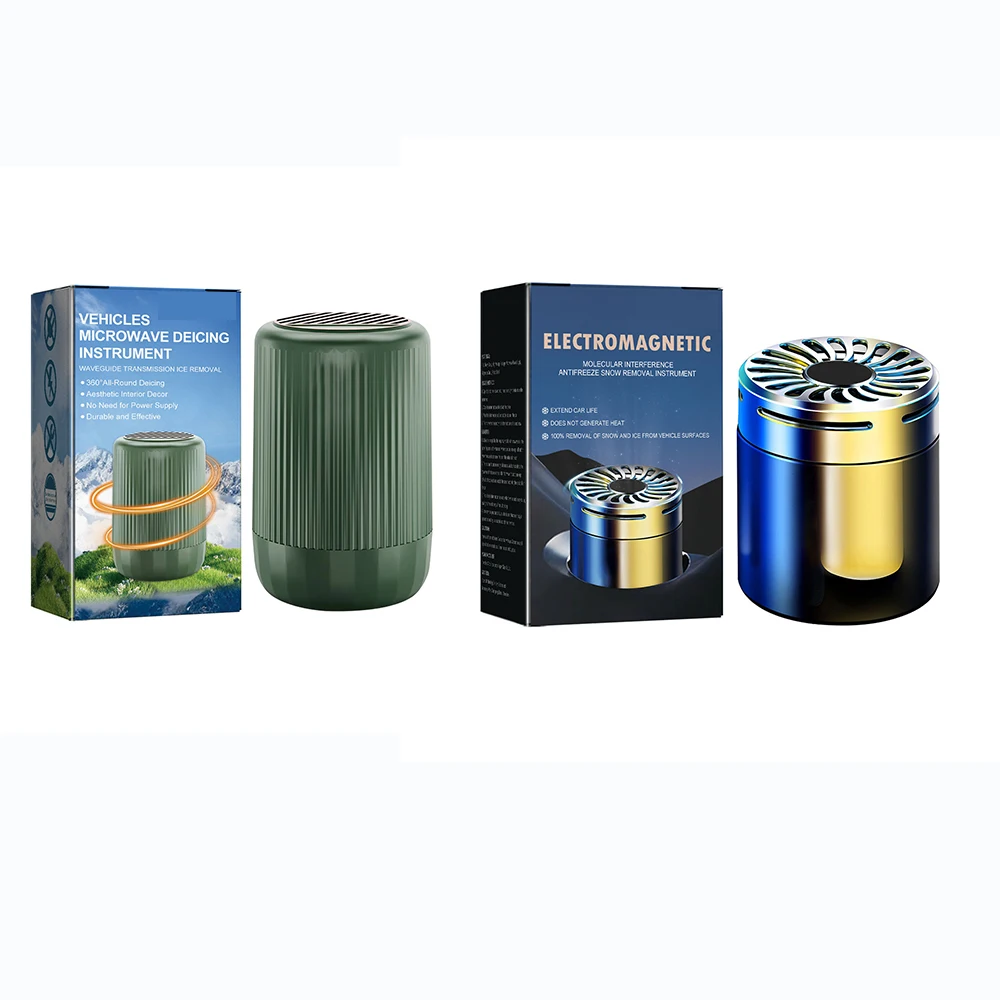The image features a detailed product listing page for microwave and electromagnetic de-icing instruments, presented in a photorealistic, landscape-oriented layout. The background is pure white, making the items and their respective packaging appear as if they are floating. On the far left is a box labeled "Vehicles, Microwave, De-Icing Instrument." It has a color photograph featuring the instrument adorned with yellow rings. To its immediate right stands the vehicle's microwave de-icing instrument itself—a tall, round, dark green canister with ridges and a vented, mesh-like top, reminiscent of a pepper shaker. To the center-right of the image, there is another box that reads "Electromagnet, Non-Cellular Interference, Anti-Freeze, Snow Removal Instrument, Extend to Car Life." This box is notably dark blue with cream-colored text. Positioned to the far right, the silver electromagnetic de-icing device reflects a blue hue. This cylindrical metal object features an open top with slits designed to allow air movement. It boasts a design that includes a screw-on top and slots to enable heat dissipation. Both devices offer different material constructions—the electromagnetic device being metallic and the microwave de-icer being plastic—providing consumers options based on preference and need.